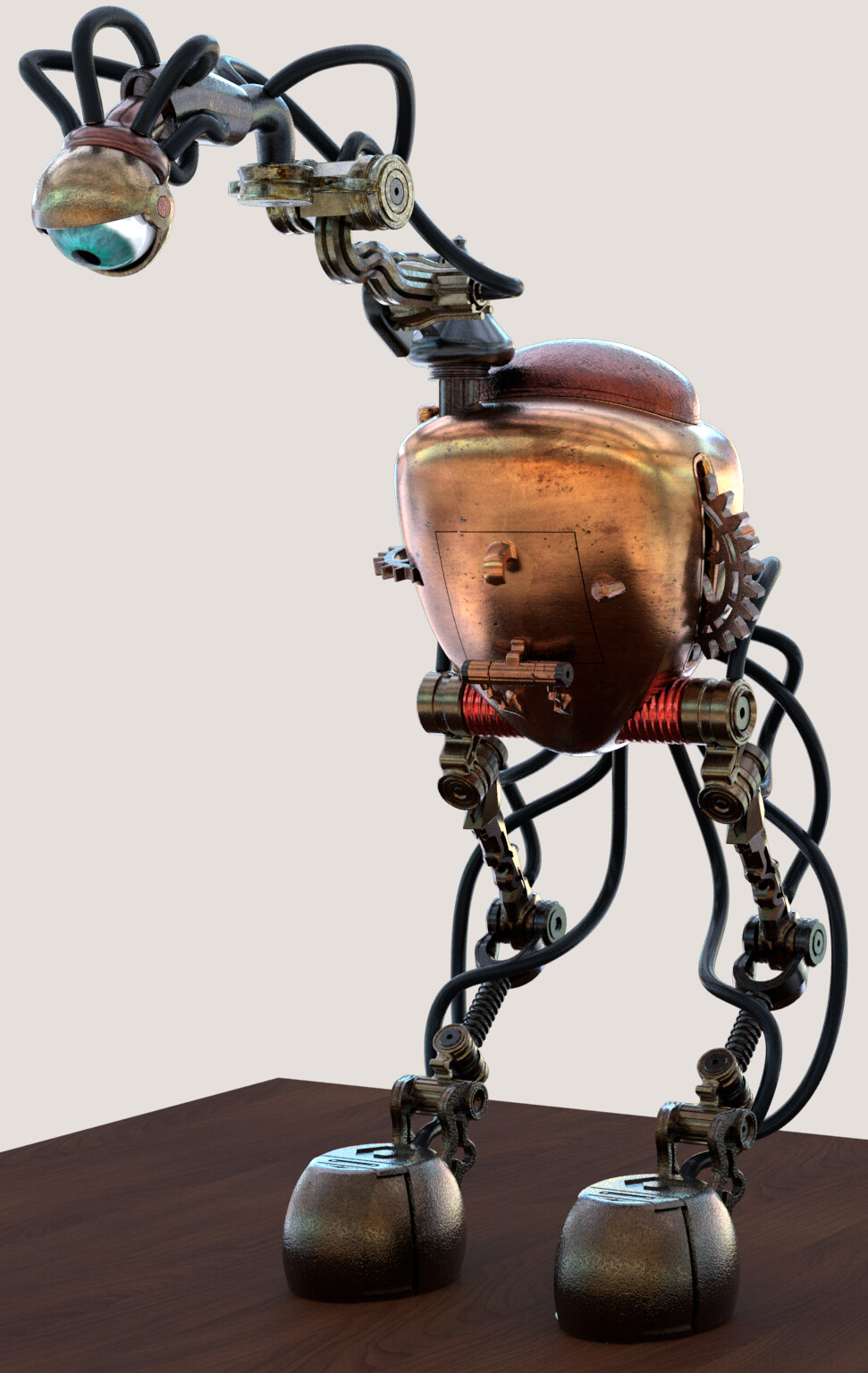In this close-up photo of what seems to be a meticulously constructed, futuristic-looking robot, the details of its metallic components are strikingly vivid. The robot has distinctive dome-shaped, dark brown feet, which appear to be heavy and crafted from iron, with legs resembling servo arms intricately folded inward, featuring interconnected wires and cables sprawling in various directions. The main body exhibits a robust brass copper color, almost like a brass container or a rounded square shape, adorned with gears on both sides. This body sits upon a red-grooved, cylindrical piece, further enriched by additional servos of a red copper hue. The neck is an intricately threaded shaft connecting to the body, culminating in a curved metal piece that supports the head. The head is essentially a singular, captivating eyeball with a blue-cyan iris, a black pupil, and a white sclera, complete with an eyelid, giving it an almost lifelike appearance. The robot is situated on what appears to be a dark orchard linoleum finish floor or possibly a solid brown wood grain desk, its realistic textures and vivid details suggesting either an actual constructed model or an exceptionally realistic drawing. The photo's close-up nature makes the robot seem almost alive, as if it could spring into action at any moment.